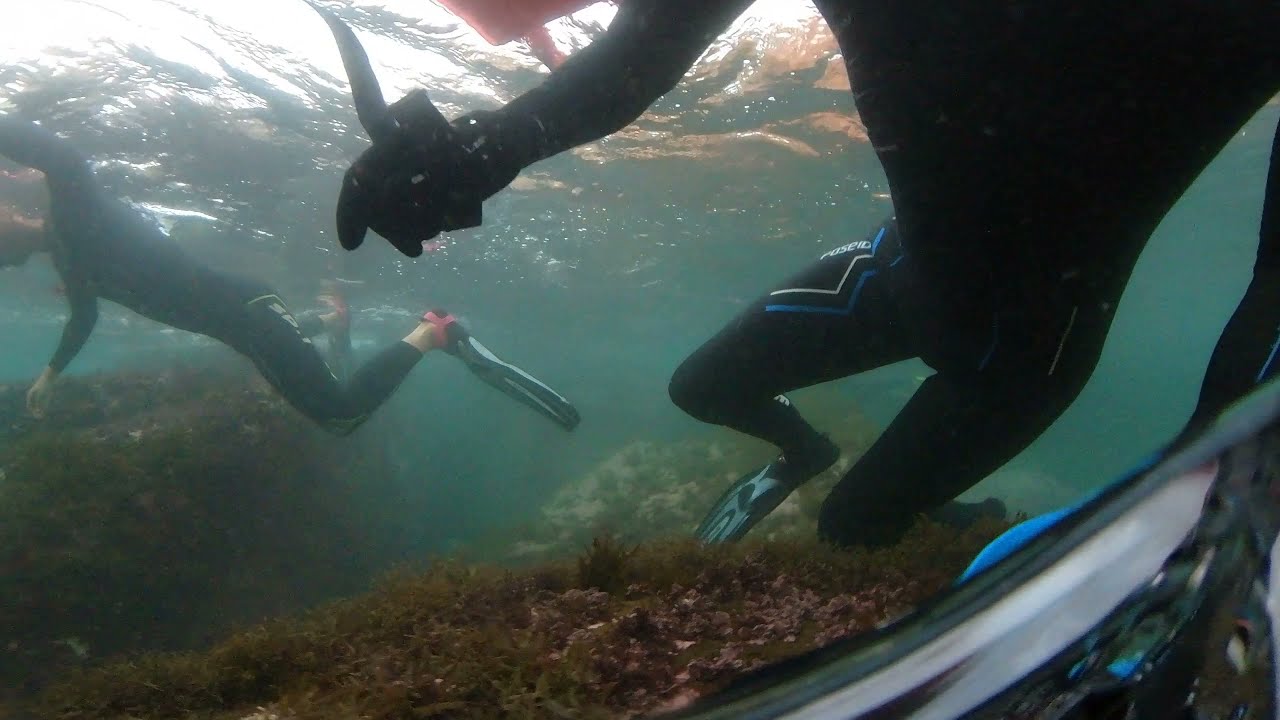In this underwater image, two people are seen snorkeling in shallow, clear blue water, captured with a selfie camera or using a fish-eye lens. Both individuals are wearing full-body black wetsuits and black flippers, with the person on the left visible from below the nose downward, showing both arms and legs. The individual on the right is visible from the chest down, holding a diving knife in their right hand. The scene is enriched with green and tan coral, seaweed, and sandy hills with green algae at the bottom. The water has a greenish-blue tint with sunlight filtering through, and a metal pole—likely part of a camera setup—can be seen in the right corner.